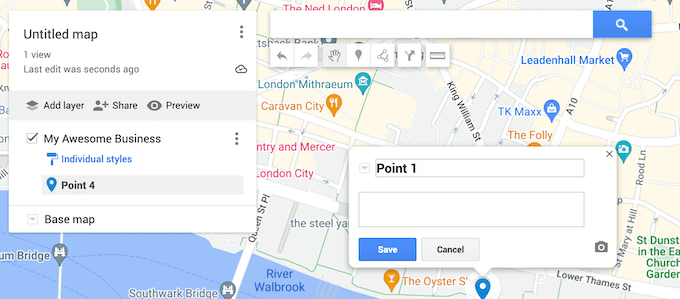A user is interacting with Google Maps, possibly located in London, though the exact location is uncertain. The map display includes the word "London," but additional context is needed to confirm this. On the left side of the interface, there is a small section labeled "untitled map," which is noted to have been edited just moments before. The user is in the process of adding a point of interest titled "My Awesome Business."

To the right of the screen, the user is further editing a label identified as "Point 1," where they can input additional details and then save the changes. The map's interface also features a search bar at the top, with various buttons beneath it. These buttons allow users to pan, zoom, highlight different points of interest, share the map, and potentially create custom routes.

In the lower left part of the screen, there is a visible body of water, intersected by multiple bridges, including the Southwark Bridge. This area provides further geographical context to the map's location, likely confirming it as London.